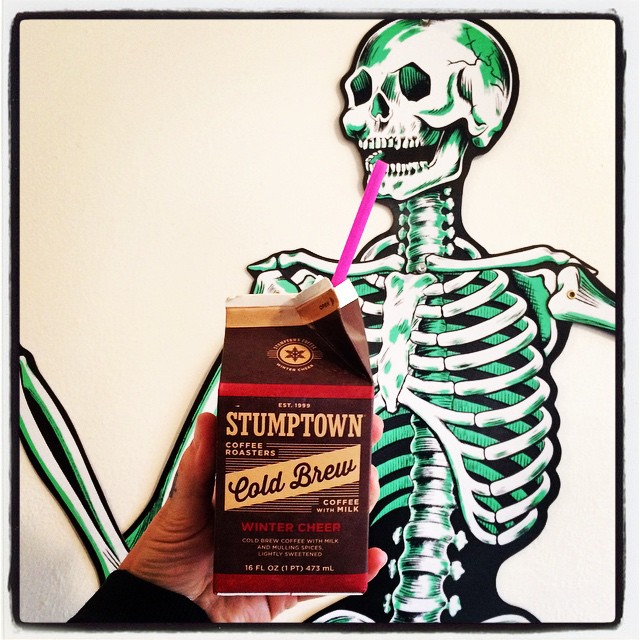In the image, there is a detailed artistic rendering of a human skeleton, set against a plain white background with a black border. The skeleton, colored white with green and black accents, appears to have its mouth slightly open and arms raised. The top half of the skeleton is visible, extending to just below the ribs. Notably, the right side of the skull has a small crack. The backdrop hues the bones green, whereas the visible ribs and neck vertebrae are white. 

In front of the artwork, a real-life fair-skinned left hand is holding a carton of Stumptown Cold Brew Coffee. This hand has noticeable creases and a tattoo on the thumb, peeking out from a sleeve of black fabric. The carton, resembling a traditional milk carton style, is mostly brown with red and yellow text. There is a purple straw protruding from the open top, directed towards the skeleton's mouth, attempting to create the illusion that the skeleton is drinking from it.

The carton features several inscriptions: "Established in 1999, Stumptown Coffee Roaster's Cold Brew Coffee with Milk," "Winter Cheer," and "Cold brew coffee with milk and mulling spices, lightly sweetened." Additional smaller text notes "16 fluid ounces, One Pint, 473 milliliters." The red text towards the bottom of the carton provides supplementary details but remains too small to discern clearly.